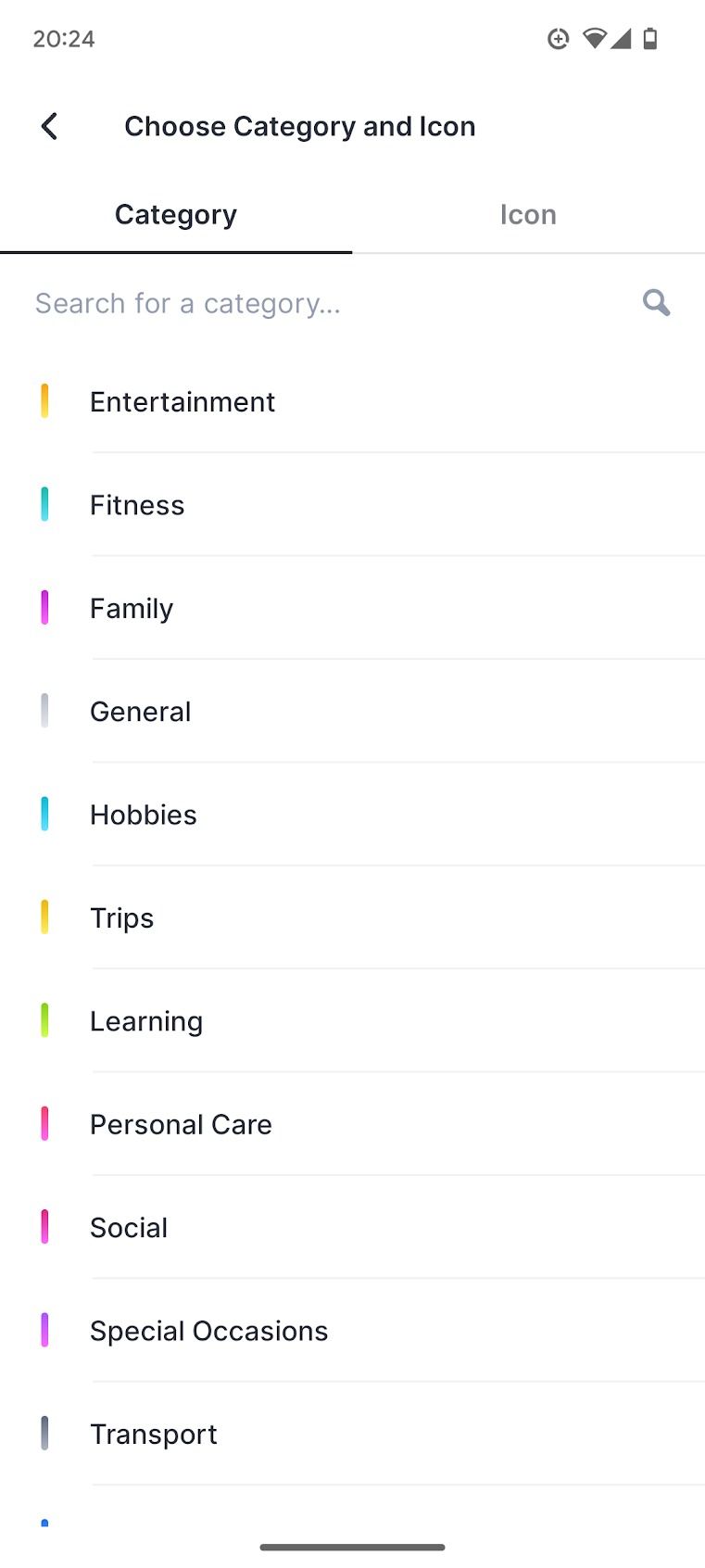The screenshot depicts a segment of a computer interface. At the top-left corner, the time is displayed as "2024 20:24". The top-right corner features several computer icons, including one indicating power and another showing battery strength. Below this, there is a gray arrow pointing to the left, accompanied by the text "Choose category and icon". 

Underneath, there are two columns: the left column is titled "Category" in bold, underlined black text, while the right column is labeled "Icon" in gray, underlined text. Below this, there is a search bar labeled "Search for a category".

Vertically aligned under the search bar are labels representing different categories, each indicated by a vertical colored line to the left of the text. The categories are as follows:
- "Entertainment" with a yellow line.
- "Fitness" with a blue line.
- "Family" with a purple line.
- "General" with a light purple line.
- "Hobbies" with a blue line.
- "Trips" with a yellow line.
- "Learning" with a green line.
- "Personal Care" with a red line.
- "Social" with a pink line.
- "Special Occasions" with a purple line.
- "Transport" with a gray line.

Below these categories, there is a blue dot, followed by a black horizontal line running across the center of the interface, which is set against a white background.